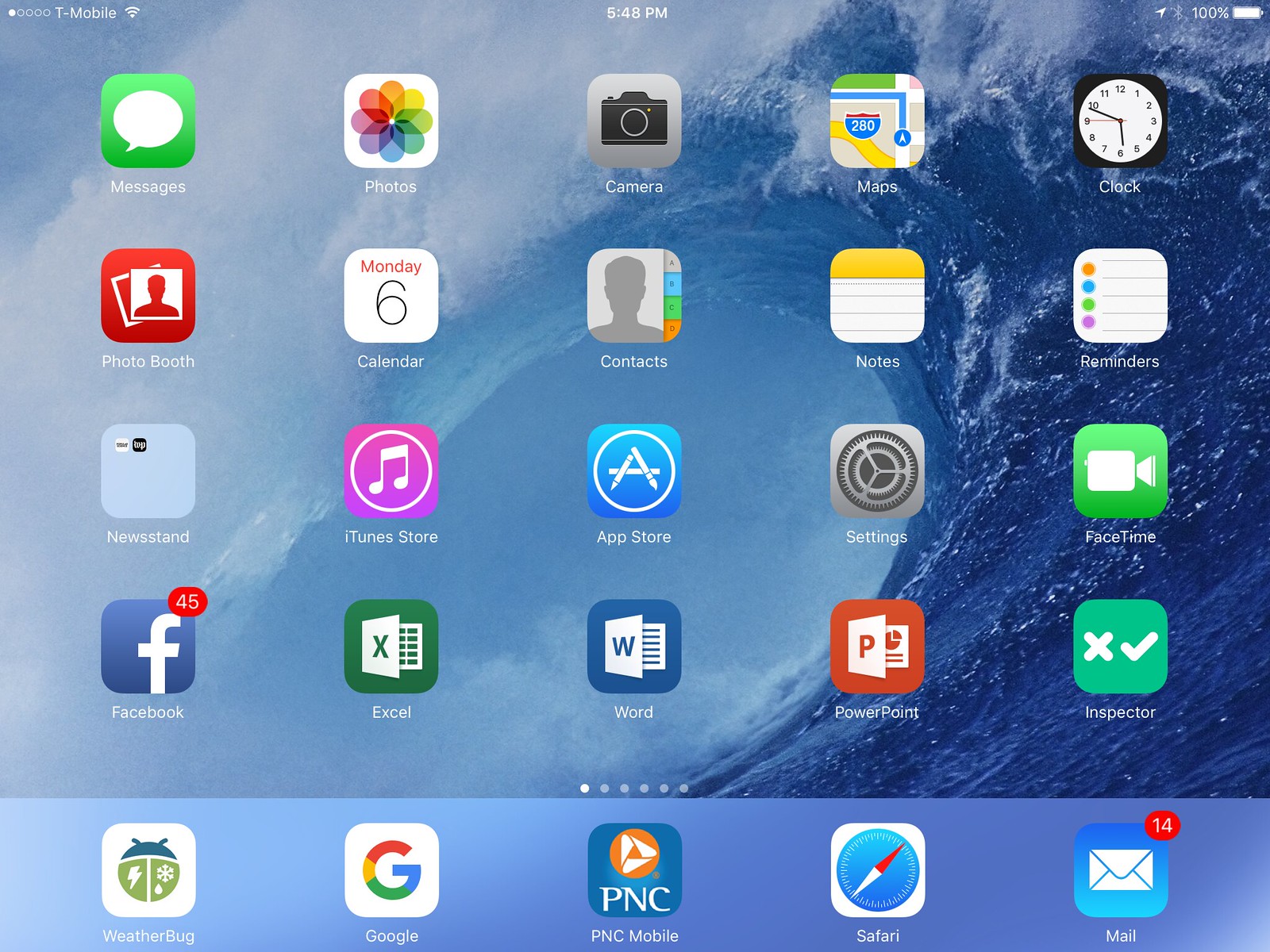This image captures a screenshot from a smartphone's home screen. Starting from the top left corner, there is an array of circles indicating cell signal strength, with only one circle filled, suggesting low signal. Beside that is the label "T-Mobile," followed by a tornado icon symbolizing a connected WiFi network. Centrally positioned at the top is the time, displayed as 5:48 PM. On the top right corner, notification icons include a triangle, representing active location services, a Bluetooth symbol, and a fully charged battery at 100%.

The background wallpaper showcases an impressive blue ocean wave, elegantly curling and cresting as if about to crash onto the shore. The home screen layout reveals that the user has multiple pages of apps, indicated by a series of dots near the bottom of the screen. We are viewing the first page, which arranges apps in a grid with five rows and five columns, forming a neat and organized display.